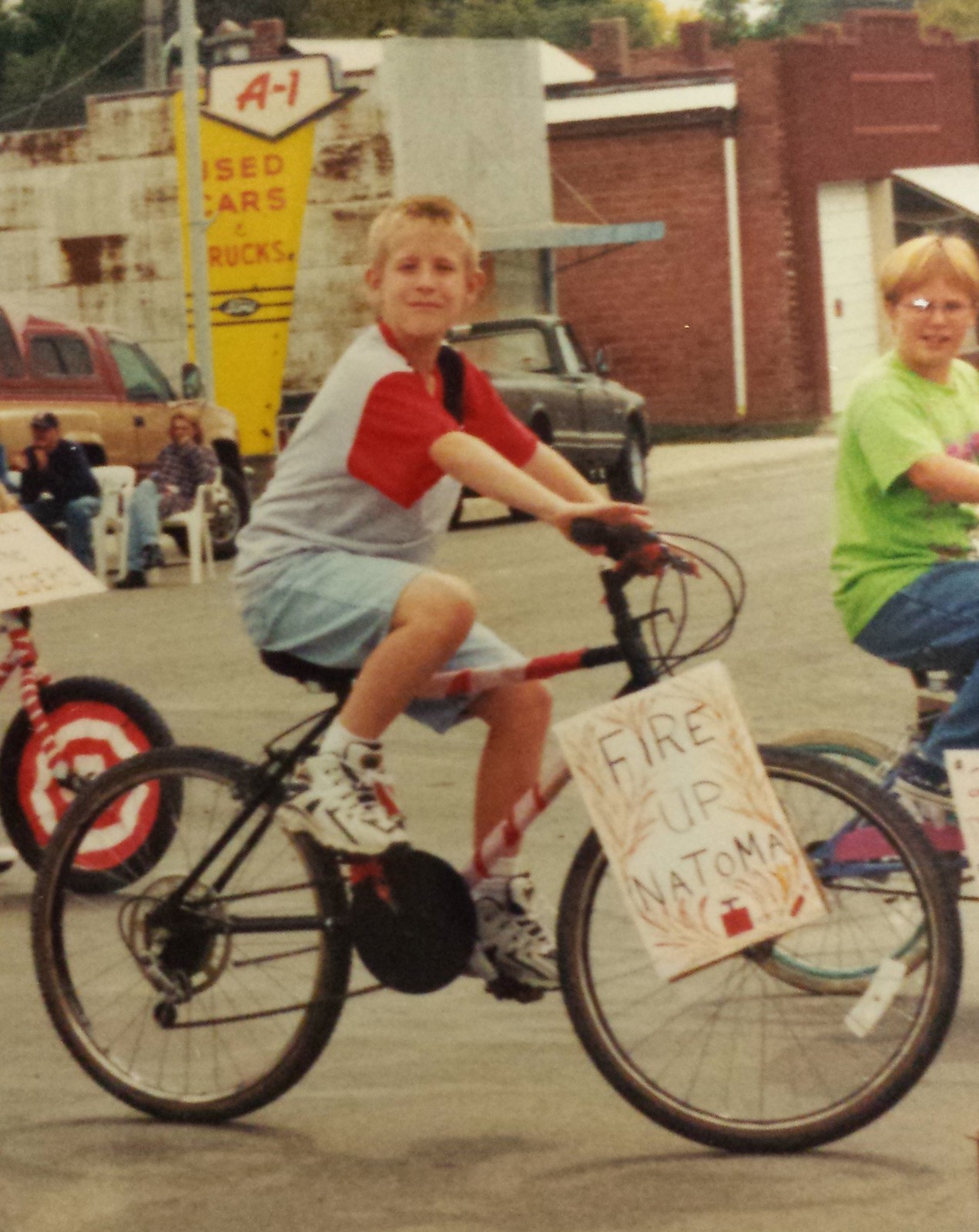The image is a color photograph with a vintage feel, possibly from the 1960s or 70s, depicting children riding bicycles in a small town setting. The main subject, a young boy about seven years old, has short blonde hair and is looking over his right shoulder towards the viewer. He is dressed in a gray t-shirt with a red collar and red sleeves, jean shorts, and white tennis shoes with black details. He rides a black bicycle with red detailing, which features a white paper sign on the handlebars that reads "Fire Up Natoma" with an illustration of fire, a stick of dynamite, and an igniter.

To the right of the central boy is another young rider, partially cut off in the image. This boy has blonde hair parted down the center, wears a green t-shirt, glasses, and blue jeans. The wheel of his bike is decorated with red and white swirls. 

In the background, there are people seated on white chairs outside a building adorned with a banner that reads "A1 Used Cars and Trucks." The photo's portrait orientation and the detailed elements provide a glimpse into the nostalgic scene, capturing the essence of a bygone era.